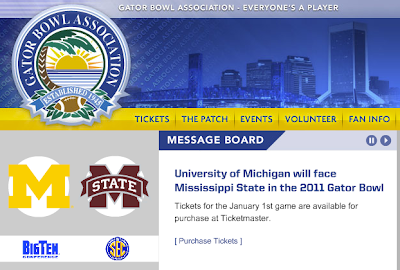The image showcases a busy webpage for the Gator Bowl Association. In the upper left corner, there's a circular logo. The text "Gator Bowl Association" wraps around the top and sides of the logo, which also features a palm tree in the center with a football at the bottom.

To the right of the logo, there's a city skyline, presumably the location for the event. Below the skyline, there is a yellow banner containing menu options such as Tickets, Events, Volunteer, and Fan Info.

Further down, there is a message board. The first message announces, "University of Michigan will face Mississippi State in the 2011 Gator Bowl." On the left side of this message board, logos for the University of Michigan and Mississippi State are displayed, with text indicating "Big Ten" under Michigan and "SEC" under Mississippi State.

At the top of the webpage, a banner reads, "Gator Bowl Association - Everyone's a player."